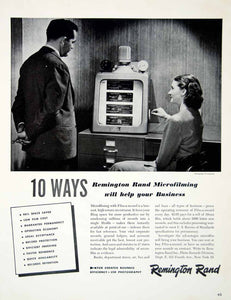This detailed black-and-white advertisement from what appears to be an old magazine, likely from the 1960s, highlights the "10 ways Remington Rand microfilming will help your business." The top half of the ad features an image of a man in a business casual suit standing to the left. He oversees a woman who is seated at a desk chair to the right. Both are engrossed in a microfilming machine that sits on the desk, likely a device for developing film. The woman has her back turned partially toward the viewer, looking up at the man with a smile as she spins a dial on the machine, suggesting an interaction that conveys the operation of the device. The background features pleated wood linoleum-like wallpaper, adding to the vintage office ambiance. Below the imagery is a list of ten benefits of the microfilming service, though the text remains largely illegible. The overall presentation exudes a professional mid-20th-century office setting aimed at promoting microfilming technology as an efficient business tool.